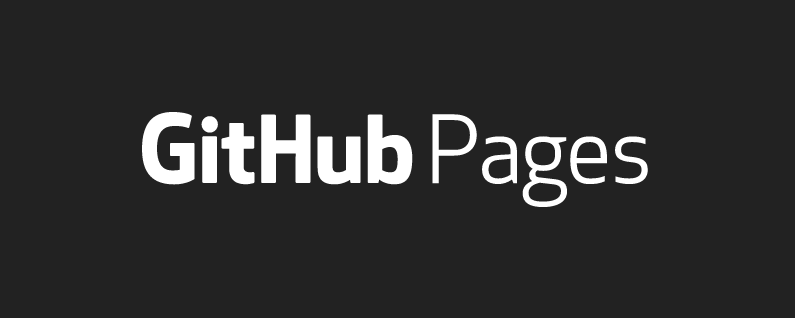This image features a minimalistic design likely intended for use as an advertisement or banner. It has a narrow, horizontal rectangular shape with a solid black background. On the left side, the word "GitHub" is prominently displayed in very bold, white text with both the 'G' and 'H' capitalized. On the right side, the word "Pages" is also in white, but in a much thinner, typewriter-style font. Both words are center-aligned within the image. There are no additional elements such as URLs, logos, or shadows, making the composition very clean and straightforward. The simplicity suggests it is a generic, versatile graphic that can be adapted for various promotional uses, whether online or in print media.